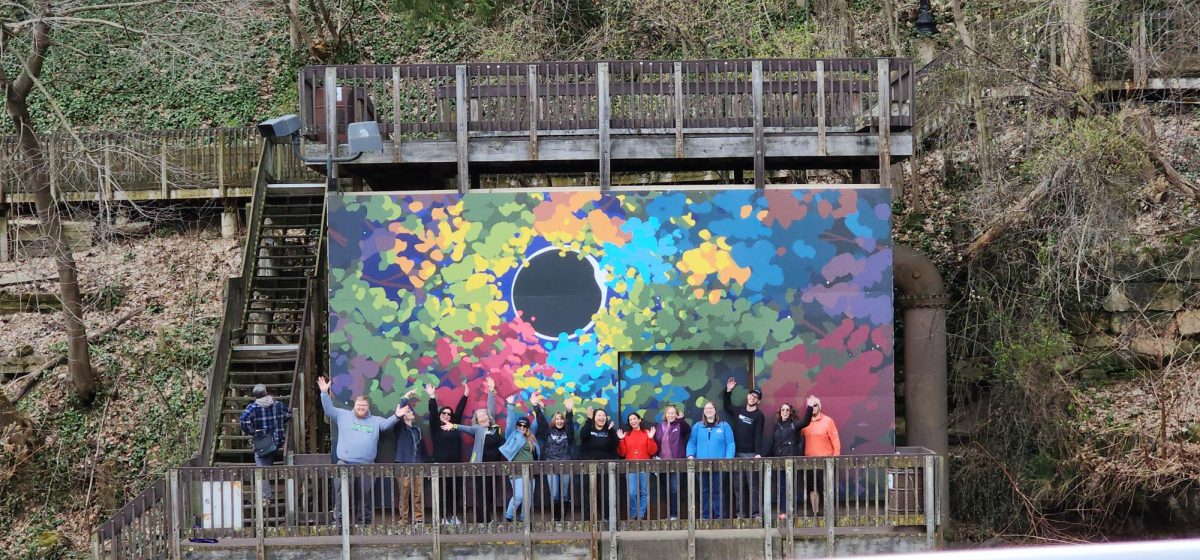This image captures a lively group of 14 people posing on a hillside adorned with greenery and interspersed with some deadfall and unhealthy trees. The scene features a gated walkway built into the hill, with an overlook at its center and stairs leading down to an additional observation deck. A prominent, colorful mural forms the backdrop, painted with vibrant blues, reds, yellows, and purples in an abstract foliage design. All the individuals in the photo are smiling and waving their hands in the air, with several displaying exuberant gestures, giving the impression of an action shot. Most are clad in cold-weather attire, including sweatshirts and jackets. Off to the left, one person is ascending the stairs, carrying a computer bag. The group's surroundings, filled with trees, vines, and bushes, enhance the outdoor wilderness vibe of the setting.